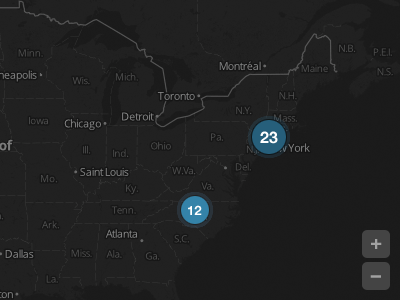The image displays a map on a screen, featuring the northeastern region and parts of the Midwest of the United States, with a portion of Canada visible at the top. The map is somewhat dark and challenging to see clearly, but notable details stand out. A prominent bluish circle near New York contains the number "23" in white. Another similar circle appears over what seems to be North Carolina, displaying the number "12." Several major cities are labeled, including Minneapolis, Chicago, St. Louis, Atlanta, Detroit, Toronto, Montreal, and New York. The map also delineates various states within this geographical area, such as Ohio, West Virginia, Virginia, Kentucky, Indiana, Illinois, Michigan, Wisconsin, Iowa, Missouri, Arkansas, and Mississippi.